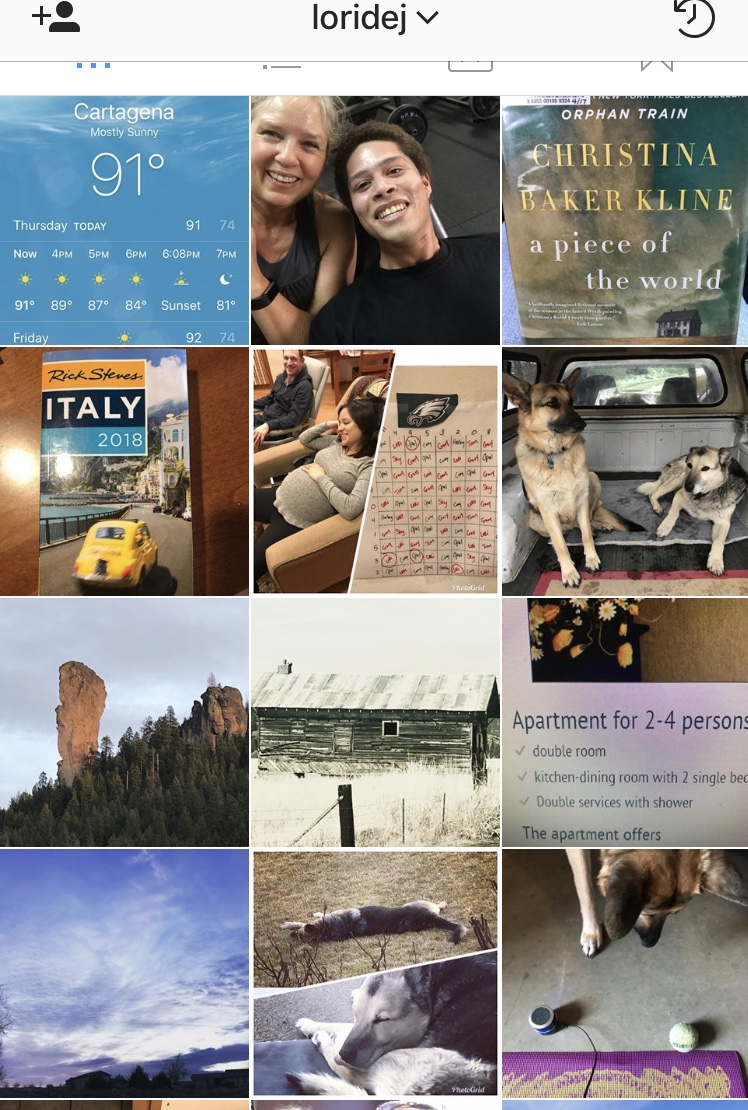Lori Desh's Instagram feed displays a curated collection of 12 images. The first photo features a screenshot from a weather app indicating the current conditions in Cartagena—mostly sunny and 91 degrees—with a forecast showing a high of 92 and a low of 74 for Friday. Next is a cheerful selfie of Lori, an older woman with blonde hair, and a man with brown hair, both smiling; Lori is dressed in a gray tank top while the man sports a black shirt. The following slide presents the cover of Christina Baker Kline's book, "A Piece of the World," depicting a solitary house in a Kansas-like field. Below this, there's a Rick Steves' "Italy, 2018" tour guide book lying on a table. The feed also includes three adorable photos of dogs, juxtaposed with a couple of scenic shots capturing the sky and mountain landscapes.